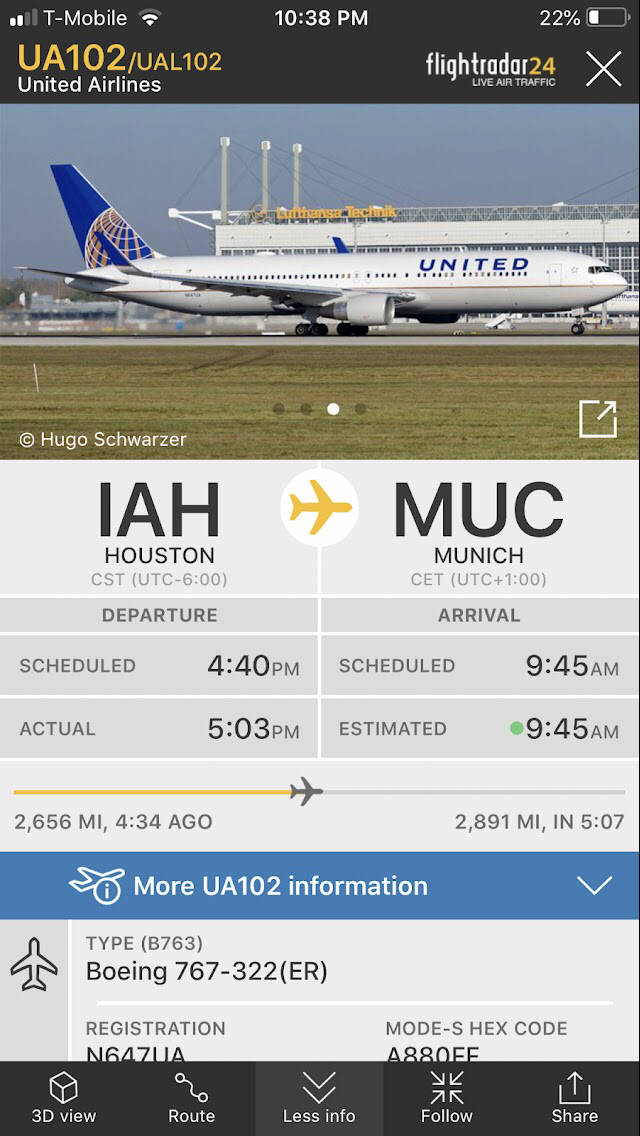On a cell phone screen, visible in the top left corner are the words "T-Mobile," indicating the service provider, alongside symbols for phone signal strength and a low Wi-Fi signal. At the center of the screen, the time reads 10:38 AM, while the battery level is 22%. The background of the screen is predominantly black, featuring the text "UA102 / UAL102" in orange at the center, under which "United Airlines" is written in white.

Prominently displayed is a white United Airlines plane on a runway in daylight, with visible airport structures and green grass around. The aircraft is branded with "United" in blue on its fuselage and has a blue tail with a globe emblem.

Above the image reads "Flightradar24" where "Flightradar" is in white and "24" in orange, denoting a live air traffic tracking application. There's a big white "X" in the top right corner of the app screen.

Below the airplane image, it reads "photographer: Hugo Schwazer," with four dots marking possible image views; one of these dots is highlighted in white, indicating the current selection.

Details about the flight are provided: the plane is departing from IAH (George Bush Intercontinental Airport in Houston) at 4:40 PM Central Standard Time (CST) [UTC-6:00] and arriving in Munich (MUC) at 9:45 AM Central European Time (CET) [UTC+1:00]. There are gold-colored airplane icons in white circles, indicating departure and arrival points. The scheduled departure and actual departure times are 4:40 PM and 5:03 PM, respectively.

Flight information includes the total distance of 2,656 miles and an elapsed time of 4 hours and 34 minutes since departure, with 2,891 miles to go and an estimated arrival time of 9:45 AM. It specifies the aircraft as a Boeing 767-322(ER), registration N64ZUA, and Mode S hex code 8880FF.

The screen also features a gray information box at the bottom, providing options such as 3D view, route details, less info, follow, and share.